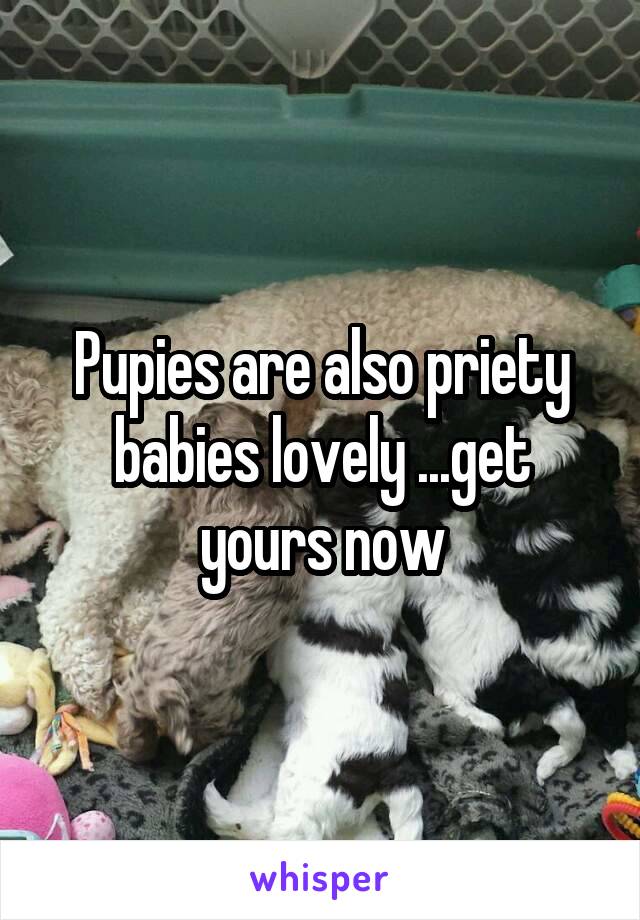The photograph depicts a scene of a mother dog, resembling a curly-haired blonde Goldendoodle, nursing a group of puppies. The mother dog lies across the center of the image, with her head on the left and her tail on the right. The puppies, predominantly black and white with one brownish puppy, are clustered towards the bottom of the image. They are within a turquoise-colored crate or container, which has a gate visible behind it. At the top of the image is the edge of a green plastic crate. Superimposed text, in bold white letters, reads: "Puppies P-U-P-I-E-S are also pretty P-R-I-E-T-Y. Babies lovely... get yours now." Additionally, the word "Whisper" is prominently displayed in purple lettering at the bottom of the image. The varied colors within the photo include different shades of gray, black, green, tan, pink, purple, orange, and yellow. The setting appears somewhat staged, suggestive of a meme or social media advertisement aimed at promoting the sale or adoption of puppies.